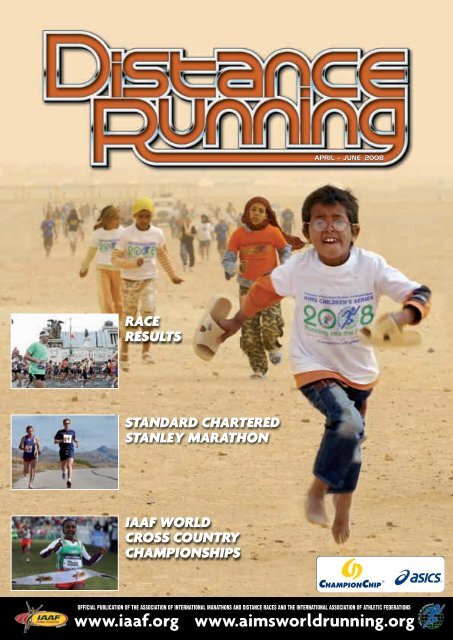The cover of the magazine "Distance Running" for April-June 2008 features a striking scene of children running barefoot through a sandy, low-visibility environment, possibly a desert. The title "Distance Running" is prominently displayed in orange text at the very top, with the extended leg of the 'R' forming part of the 'G'. Below this, in white text, is the publication date. On the left side of the cover, text highlights include "Race Results," "Standard Chartered Stanley Marathon," and "IAAF World Cross-Country Championships." The image background shows several children, one in particular wearing glasses, jeans, and no shoes. Additional images to the left depict various race scenes, including runners in different landscapes and a woman wearing a number. At the bottom right, logos for sponsors like ASICS, IAAF, and the Association of International Marathons can be seen, along with the website addresses www.iaaf.org and www.aimsworldrunning.org. The cover also mentions the publication's official status with the Association of International Marathons and Distance Races and the International Association of Athletics Federations. The color palette includes shades of white, blue, yellow, green, peach, orange, tan, and gray.